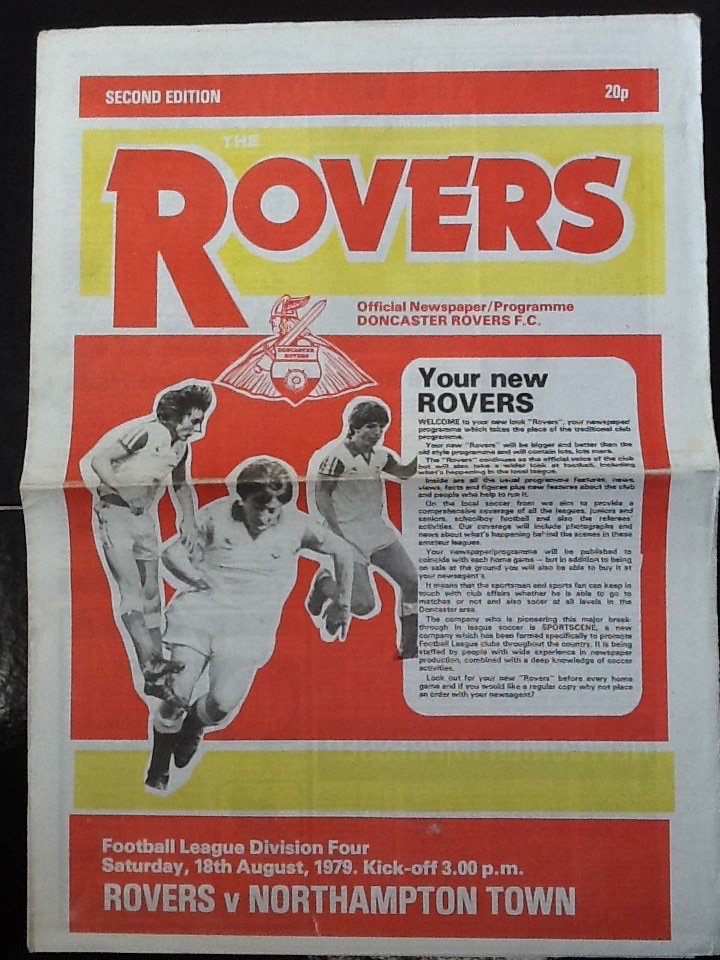The image showcases the front cover of the Doncaster Rovers FC official newspaper program from the Second Edition, priced at 20p. Dominating the top section is a red rectangular header with white text: "Second Edition" on the left and "20p" on the right. Below the header is a yellow rectangular bar with the word "Rovers" in large red letters, followed by the title "Official Newspaper/Program Doncaster Rovers F.C." Immediately below this title, the Rovers insignia is prominently displayed.

The central section features a large red rectangle, depicting three soccer players in black and white – two in the background and one in the foreground – making dynamic kicking motions. Adjacent to the players on the right side, a white vertical rectangle contains the headline "Your New Rovers" and includes an article likely introducing new team members or features.

At the bottom of the cover, a long yellow pre-footer borders a red footer which states the event details: "Football League Division Four, Saturday, 18th August 1979, Kickoff 3 p.m., Rovers vs. Northampton Town." The flyer’s distinct vintage design, with its bold red and yellow accents, ensures a striking appearance typical of 1970s sports programs.